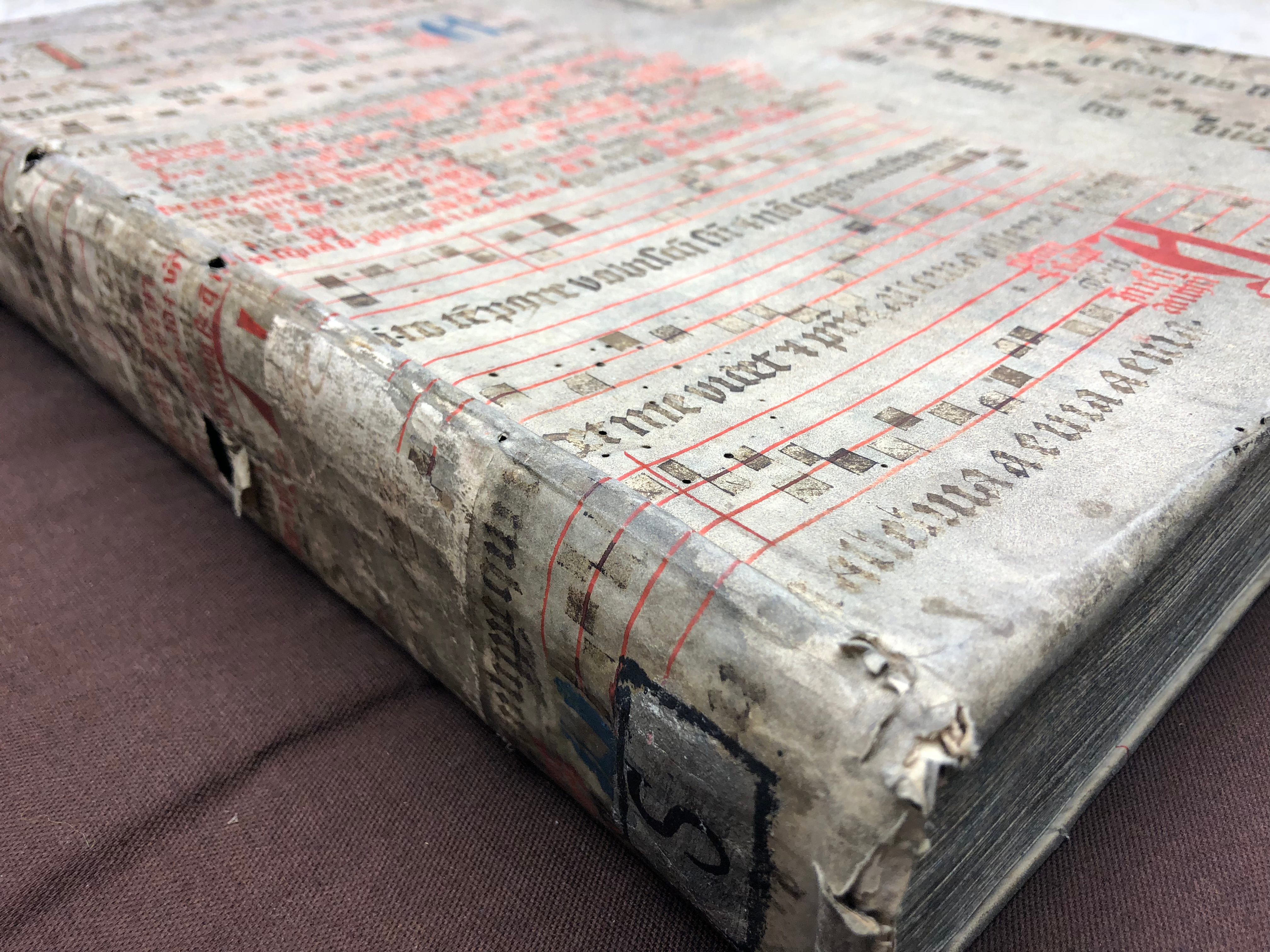The image depicts an aged and worn music book resting on a brown cloth-like surface. The book has a fragile, peeling white cover that has browned with age, particularly along the spine where there are visible tears and rips. The cover features elements of old musical notation, with four staff lines drawn in red and lacking a clef, indicating its ancient origins predating modern musical notes. Grey-gold notes and letters are scattered across these lines. Prominently, there is a large black S set against a silver backdrop enclosed in a black-trimmed box at the bottom of the cover, suggesting it might represent Volume S. Additionally, the cover displays red and dark gray or black lettering, with a conspicuous large red H. The text and notation style suggest it might be an old Latin or possibly German music book, possibly containing chant music. The overall appearance underscores the book’s considerable age and historical value.